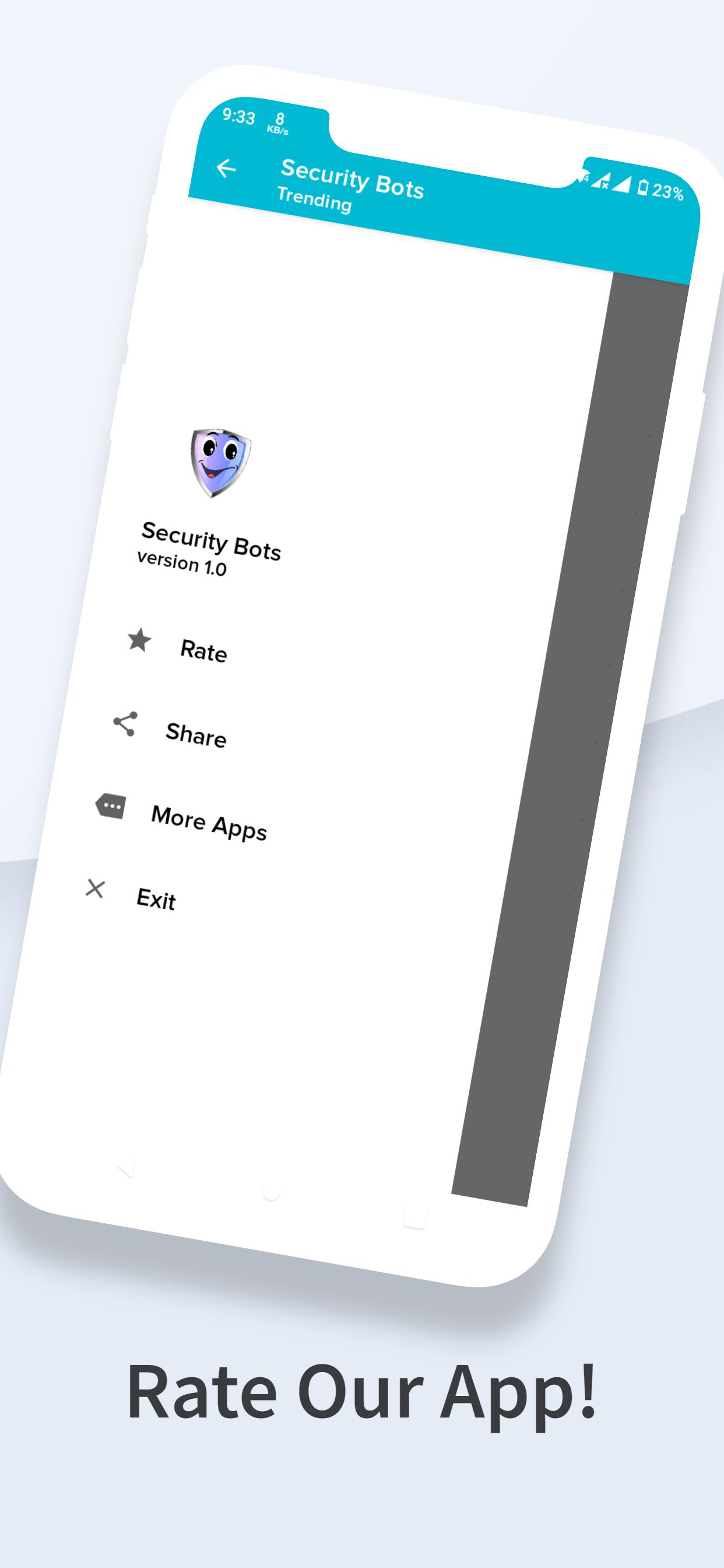The image is a promotional graphic encouraging users to "Rate our App." The background subtly transitions from white at the top to light gray at the bottom. Central to the image is the outline of a diagonally positioned smartphone screen. 

At the top of the smartphone screen, against a teal background, are various interface elements: the text "Security Bots" along with the label "Trending," the current time displayed as "9:33," and icons for Wi-Fi connectivity, signal strength, and a battery indicator showing 23% charge. An arrow pointing to the left is also visible next to the "Trending" label.

Running vertically down the right side of the phone, there is a gray rectangle. In the middle section of the phone's screen, the text "Security Bots" and "Version 1.0" are prominently displayed. Below this, icons for different actions are arranged: a star labeled "Rate," a sideways V with three dots for "Share," a ticket symbol for "More Apps," and a traditional X icon labeled "Exit." The entire composition directs attention towards engaging with the app, whether by rating, sharing, or exploring more options.